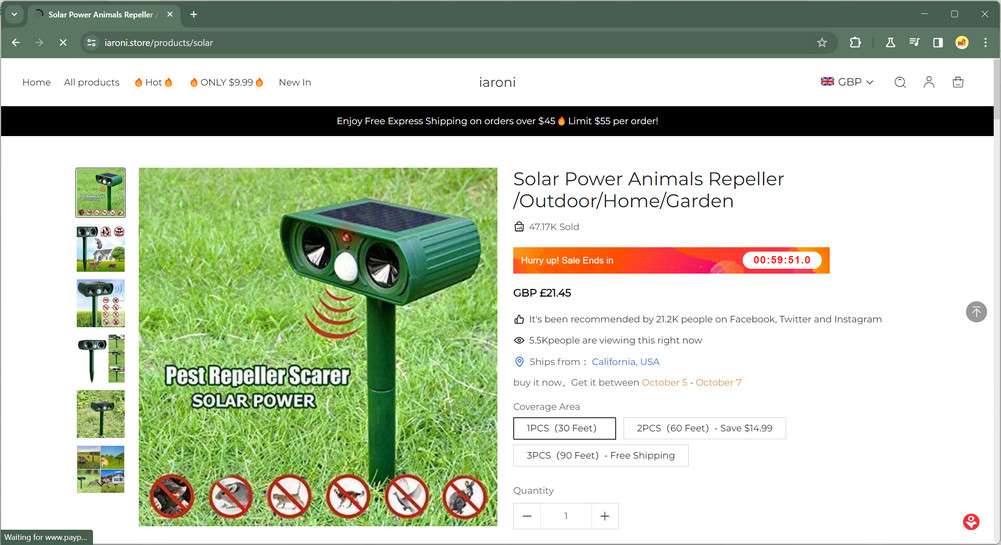Screenshot of a product page from IARONI.store showcasing a solar-powered pest repeller. The URL in the address bar is "IARONI.store/product/solar". The navigation bar lists options: Home, All Products, Hot, Only $9.99, New In, IARONE, with currency in GBP, alongside search, profile, and shopping bag icons. 

A banner below highlights "Enjoy free express shipping on orders over $45, limit $55 per order".

The main image displays a green rectangular solar-powered pest repeller mounted on a green post in a vibrant green lawn. The device features a solar panel on top and two round lenses on the front, emitting illustrated sound waves. It is labeled "Pest Repeller, Scarer, Solar Power". 

Additional images show various pests with red crossed-out signs over them, indicating the device repels moles, mice, cats, dogs, birds, and rabbits. 

A sidebar notes: "Solar Power Animals Repeller - Outdoor Home Garden. Hurry up, this item is in 59 minutes, 51 seconds". The price is GBP £21.45. The product has been recommended by 21.2K people on Facebook, Twitter, and Instagram, and is currently viewed by 5.5K people. 

The product ships from California, USA, with an estimated delivery between October 5th and October 7th. Coverage options include:
- One piece: 30 feet.
- Two pieces: 60 feet, saving $14.99.
- Three pieces: 90 feet, with free shipping. 

The quantity selected in the screenshot is one piece. A call-to-action button reads "Buy It Now".